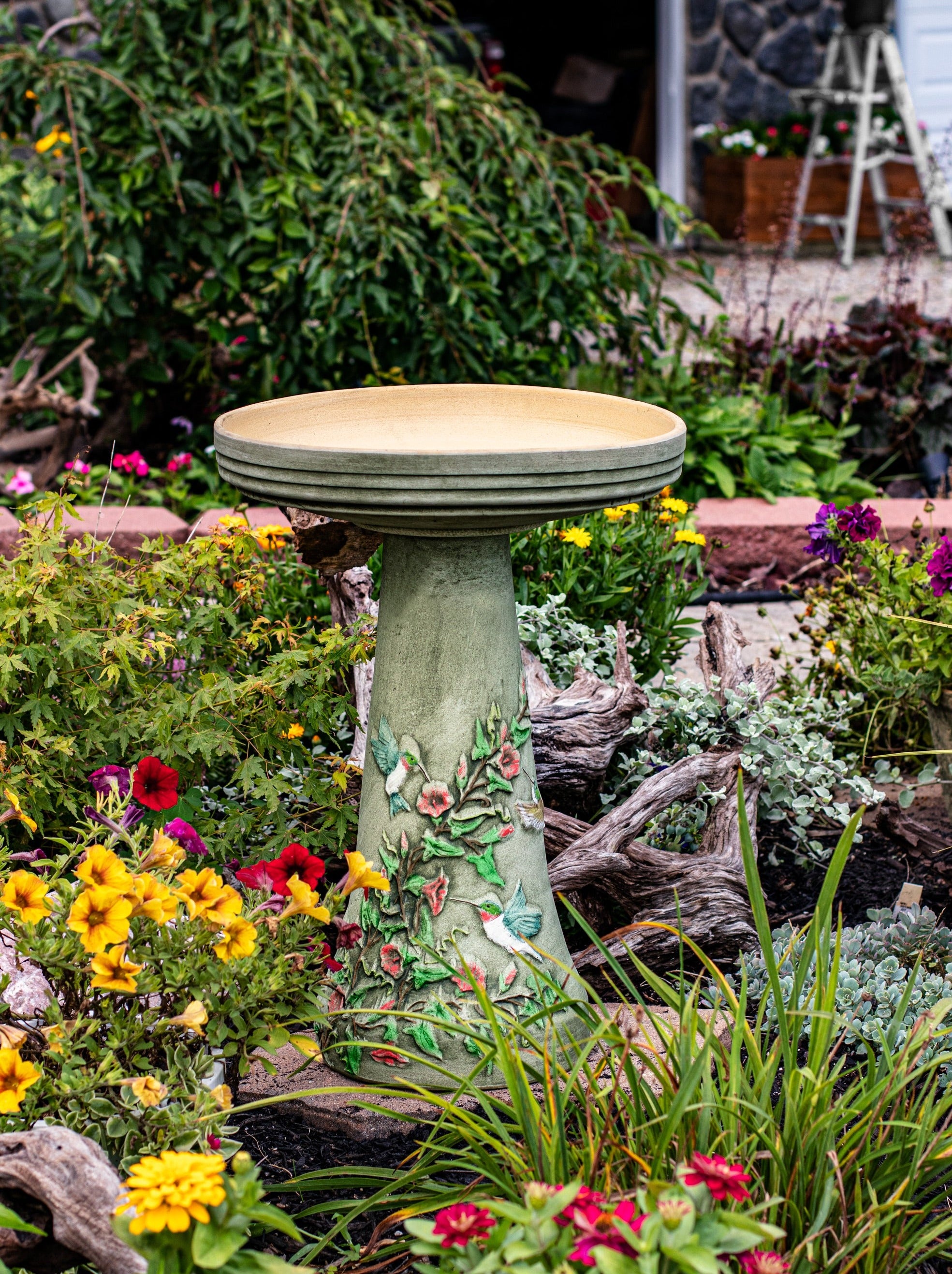The photograph captures a serene garden scene centered around a gray cement birdbath adorned with intricate designs. The birdbath features blue-winged, green-headed hummingbirds with white bodies and is embellished with red flowers and green leaves. The bowl-like top, made to hold water, invites birds to rest on its edge. Encircling the picturesque birdbath is a vibrant array of flowers, including red, yellow, pink, and purple blooms, all interspersed with rich greenery. Small stones and patches of green leaves dot the garden floor, adding texture to the scene. In the background, red bricks pave a path to another garden area where a silver ladder with a black top is set up. Beyond this, one can observe green grass, bushes, and a combination of cinder block and wooden structures, further enriched by flowers of various colors. An open door adds depth to the image, along with overgrown green bushes in a distant corner. The overall composition of the garden offers a peaceful contrast between the carefully crafted birdbath and the lush, diverse plant life surrounding it.